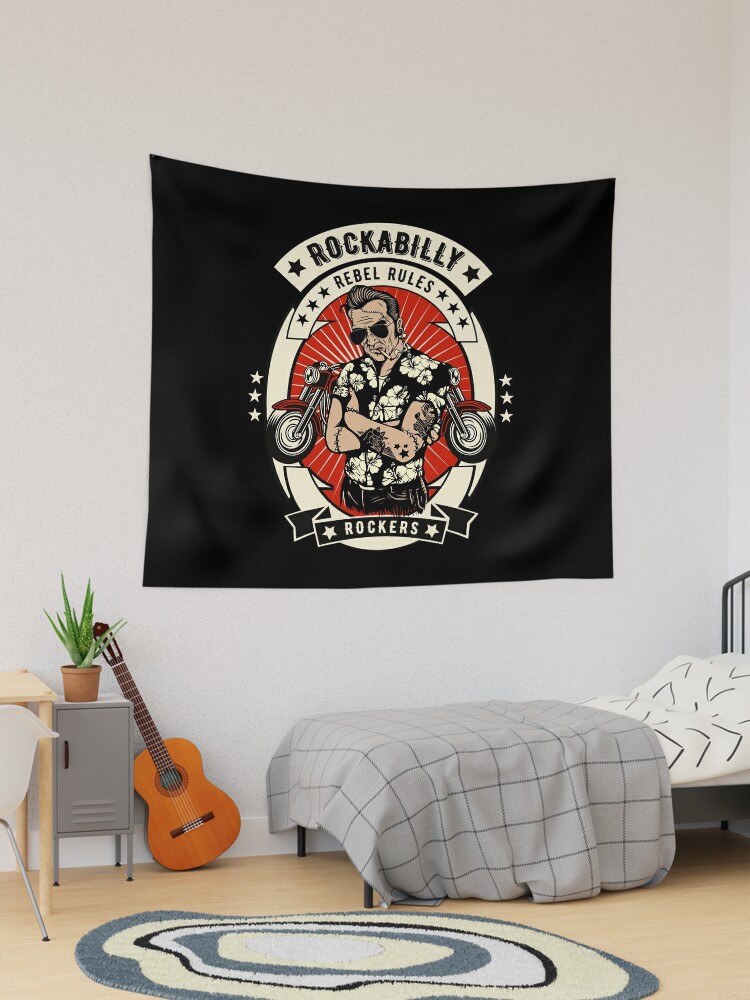This photograph captures a well-decorated bedroom with a striking centerpiece. Dominating the white-gray wall is a large, slightly sagging black banner reminiscent of a flag, depicting a stylized 1950s greaser. The central figure is a cool-looking, tattooed man with slicked-back hair, wearing sunglasses, a black Hawaiian shirt with white flowers, and smoking a cigarette. This image is flanked by two motorcycles and bordered by stars—three on each side. At the top of the banner, bold white text reads "Rockabilly," with "Rebel Rules" and "Rockers" inscribed below.

Below this eye-catching banner is a simple single bed with a black metal frame, covered by white sheets and a gray checkered quilt. Next to the bed is a gray nightstand, reminiscent of a school locker, holding an aloe vera plant on top. Leaning against this nightstand is an acoustic guitar, adding to the rock-and-roll theme. Adjacent to the nightstand is a wooden desk partially visible, paired with a white chair with metallic legs. The room’s wooden floor is partially covered by a circular rug featuring a pattern of concentric stripes in shades of gray, beige, black, and white. The overall aesthetic marries rockabilly culture with a clean, modern design, creating a unique and inviting space.